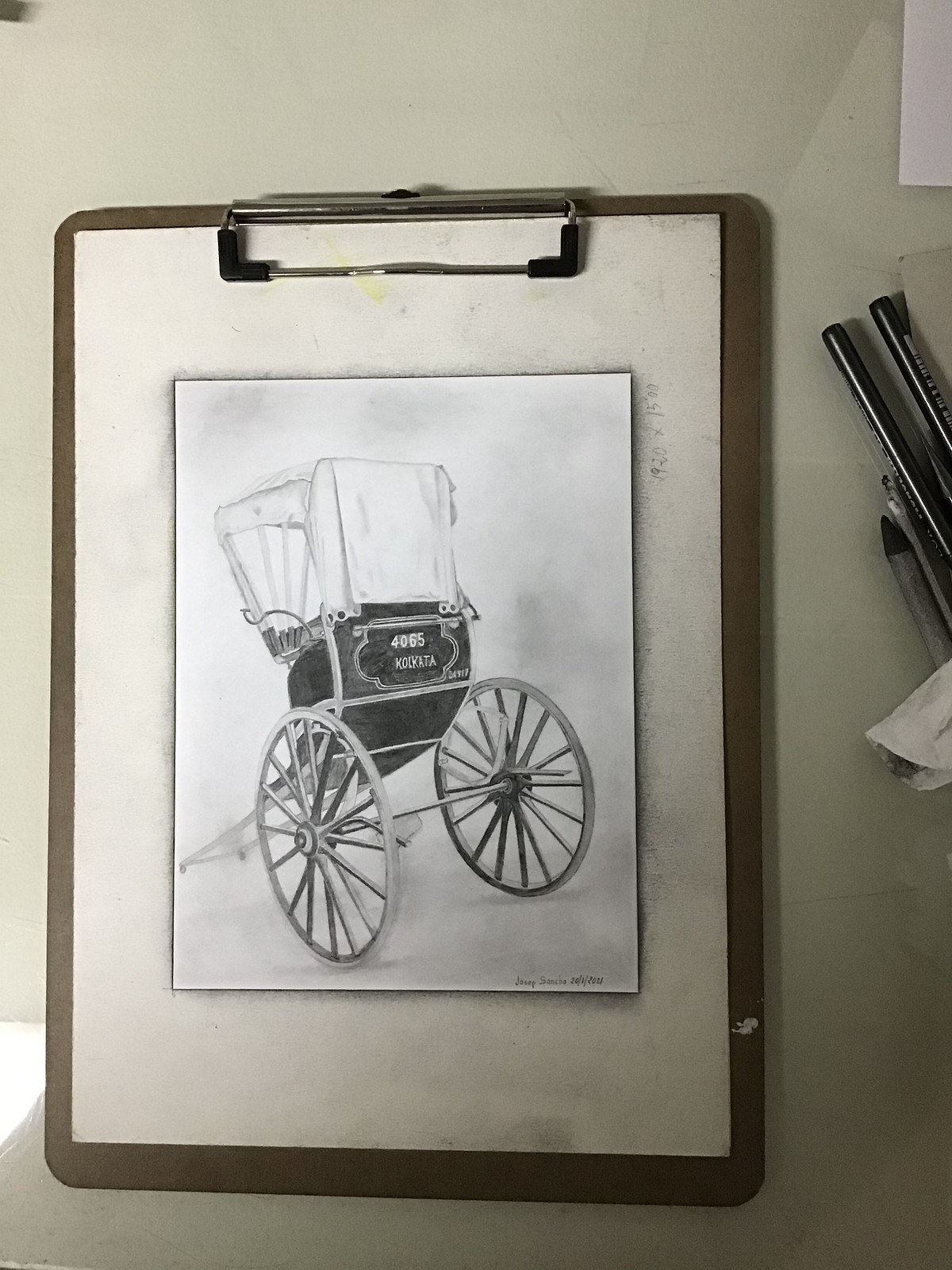The image is a high-resolution color photograph capturing a detailed scene from above. Centered on a brown clipboard with a metallic clip at the top, there is a line drawing rendered on light cream-colored paper. The drawing features an old-style wagon, reminiscent of those used by the Amish, positioned within a dark-rimmed internal triangular frame. The wagon is intricately detailed with its top section in white and the middle in black, showcasing a white logo. Two large, spoked wheels are prominently displayed, and part of the harnessing structure is visible at the left edge, indicating where it would attach to a horse. Surrounding the drawing, in the upper right-hand corner, lie the edges of two black pens along with some scraps of paper. A light shadow is cast towards the lower left corner of the photograph, adding depth to the otherwise monochromatic palette that carries a subtly greyish-greenish tint.